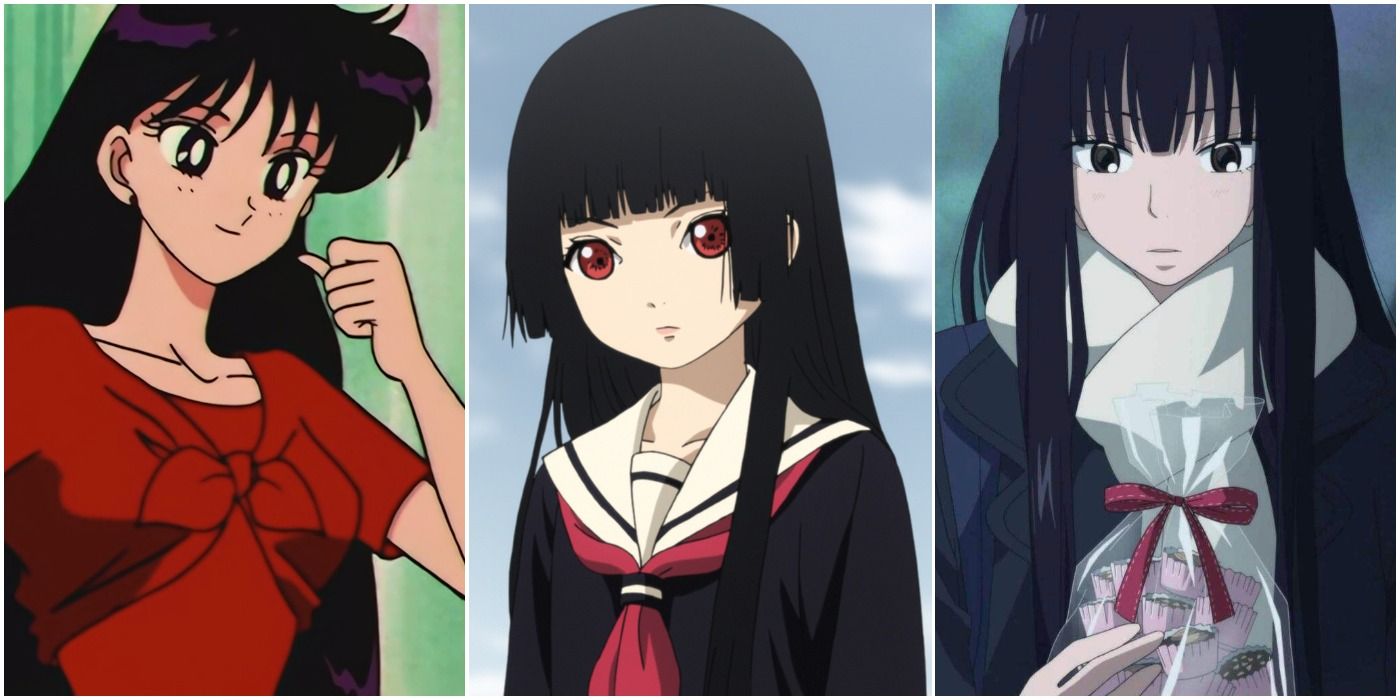The image features three anime-style girls arranged in a widescreen format, each occupying a third of the space. On the left, a determined-looking girl with long black hair and large eyes stands with her left fist clenched. She is wearing a red dress tied with a ribbon at her chest, sporting white eyes with black irises and a white pupil. The middle section showcases another black-haired girl with striking red eyes and pale skin, dressed in a dark sailor school uniform with a white collar and a red tie. She looks serious and composed. On the right, a girl with long black hair and grayish-black eyes is dressed in a blue coat and white scarf. She is holding a clear cellophane bag with a red bow, which contains cupcakes in pink wrappers. Her expression is one of surprise or curiosity. All three girls share a somber or serious demeanor, with detailed and fine anime artistry emphasizing their unique features and attire.